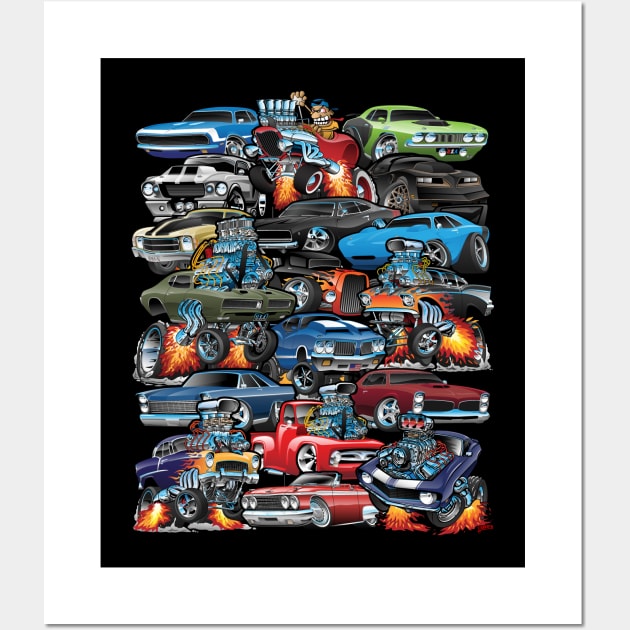The image is a vibrant and detailed poster featuring an array of animated muscle cars, predominantly hot rods and supercars, arranged in a stacked, columnar format against a solid black background. The cars are depicted in various colors – blue, green, red, gray, purple, and black – with some featuring prominent, protruding engines. Each row appears to consist of approximately three cars, stacked on top of each other, creating a visually compelling collage that echoes the aesthetic of classic muscle cars reminiscent of the Fast and Furious films. The artwork is surrounded by a white frame, enhancing its vividness against the black canvas. Among the cars, a few animated characters can be seen driving, adding a playful element to the overall composition. This eclectic collection includes models that resemble Dodge Chargers and Chevy Chevelles, with individual vehicles standing out due to their distinctive designs and vibrant colors, all contributing to the dynamic and fanciful feel of the poster.